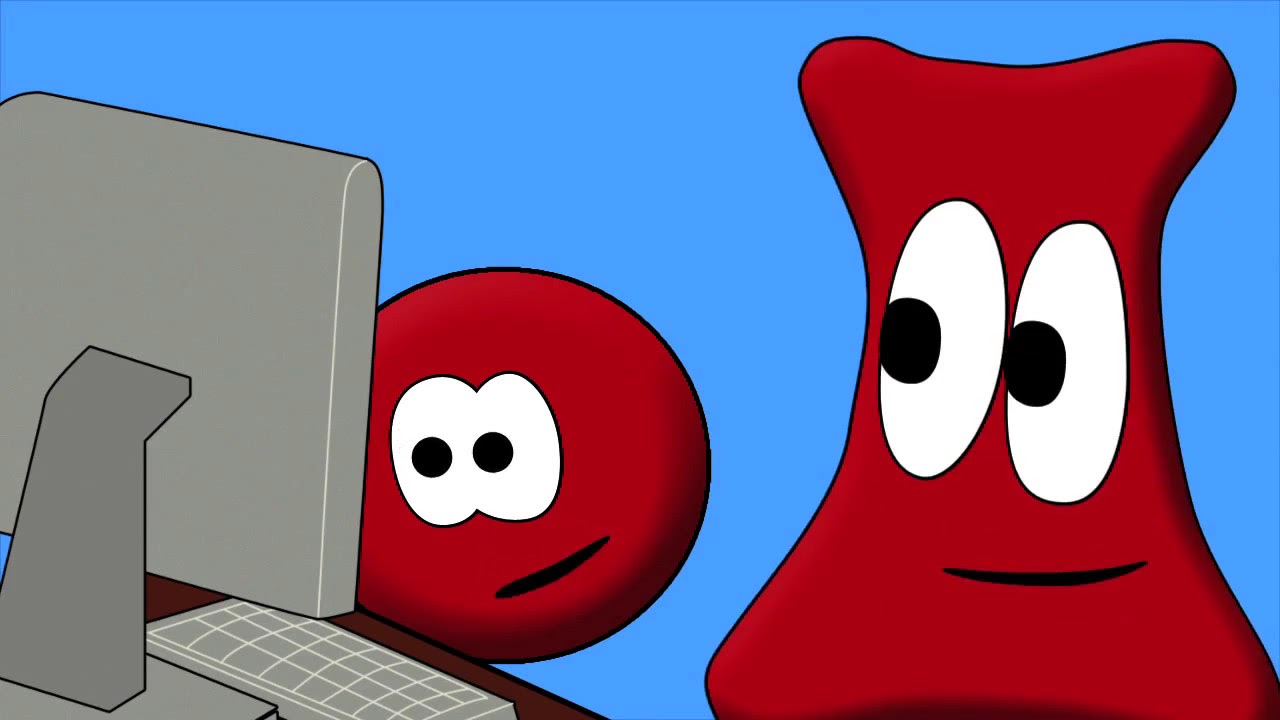In this cartoon illustration, two red animated characters are depicted against a bright blue background. The character on the left is a red circle that resembles a blood platelet, featuring large white eyes with dark brown pupils, and a mouth turned slightly upward into a subtle smile. On the right, the character is shaped like a red thumbtack or a dog bone, with a narrow center and a wider top and bottom. This character also has large white eyes with dark pupils and a slightly more pronounced smile. Both characters are intently focused on a gray computer setup with a tall monitor and a keyboard made of intersecting white and gray lines. The computer sits on a small brown desk, viewed from the back, adding to the simplicity and charm of the scene. Despite their simple design, the characters' big expressive eyes and slight smiles convey a sense of engagement and curiosity as they gaze at the screen.